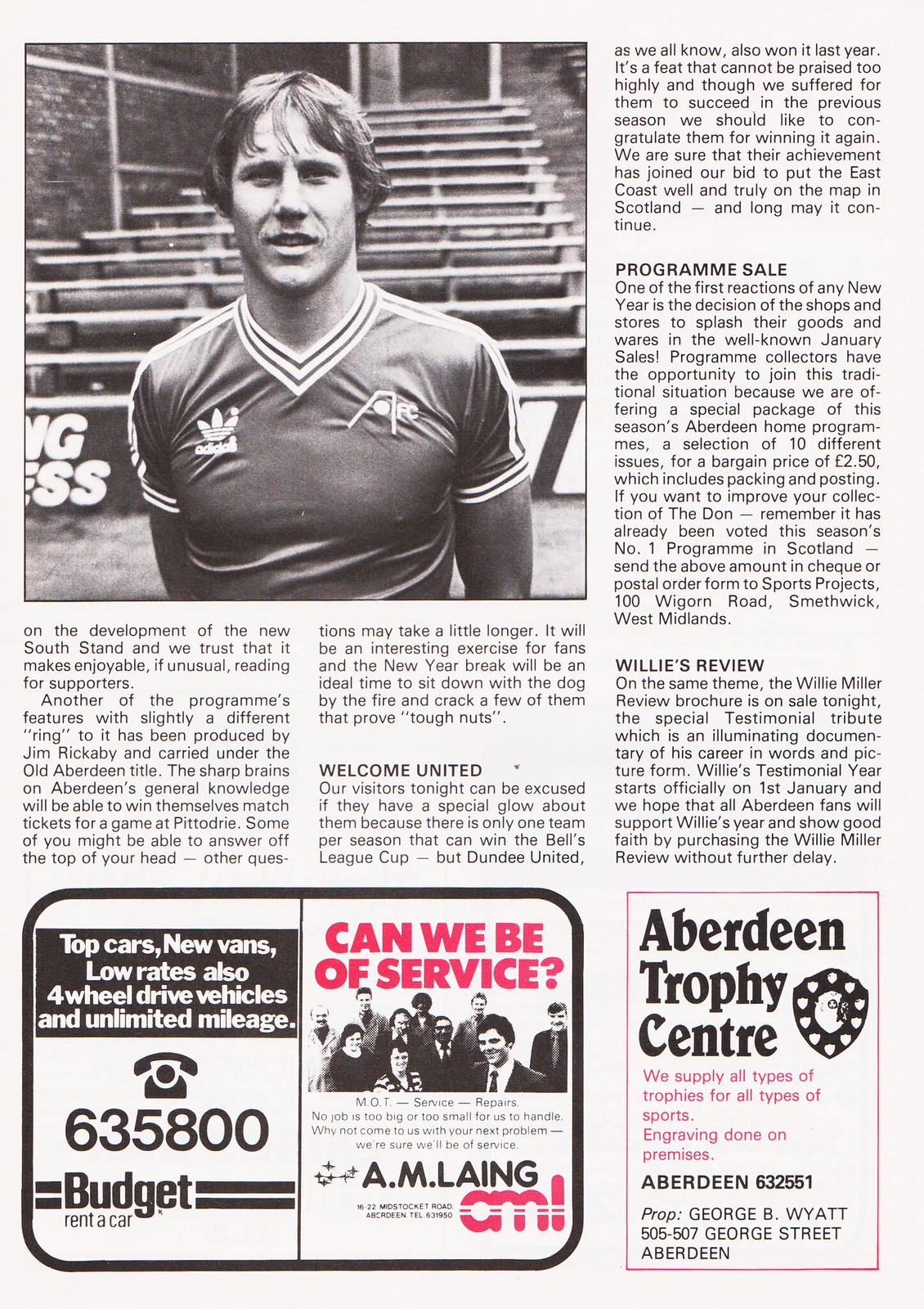This magazine or newspaper page features a prominent black and white photograph of a Caucasian man with short hair, standing in front of empty bleachers enclosed by a fence. He is wearing a v-neck Adidas jersey and has his arms positioned behind him, suggesting he might be an athlete. The high-density text of the page includes multiple article headers such as "Welcome United," "Program Sale," and "Willys Review," along with editorial content mentioning the development of the new South Stand, and program features developed by Jim Rickaby under the Aberdeen title, offering quiz opportunities for fans.

At the bottom section of the page are various advertisements. One ad from Budget Rental Cars boasts "Top Cars, New Vans, Low Rates, Also 4-Wheel Drive Vehicles, and Unlimited Mileage," with contact details listed as 635-800-BUDGET. Adjacent to this, another ad queries, "Can we be of service?" from A.M. Lange, featuring an image of people. On the bottom right-hand edge of the page, there's an ad for Aberdeen Trophy Center, which supplies a variety of sports trophies with engraving services available on the premises. Their contact number is noted as 632-551.